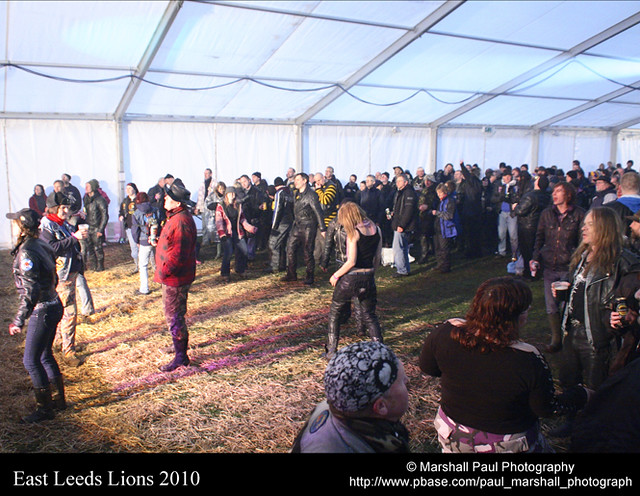This rectangular photograph, captured by Marshall Paul Photography in 2010, depicts a lively event held under a large temporary tent. The venue, possibly an indoor greenhouse, features transparent or light white ceilings, which allow ample light to filter through, and white curtains as the back wall. The structure is supported by metal poles and crisscross beams, visible at the top third of the image.

In the center of the scene stands a woman dressed prominently in black leather pants and a tight black t-shirt, appearing to either dance or stand at an unusual angle. Surrounding her is a diverse crowd of adults, predominantly in heavy clothing, including jeans, leather jackets, and boots. A man in a red jacket, red camo pants, and a hat stands nearby, adding to the vibrant mix of colors, which include shades of blue, white, red, black, and green.

The ground is a blend of yellowish dead grass or straw on the left, transitioning to greener grass on the right. People in the crowd hold drinks and look toward the left side of the image, suggesting their attention is captured by something outside the frame, perhaps a musical performance.

At the bottom of the image, a black footer with white text reads "East Leeds Lions 2010" on the lower left. The right corner bears the copyright mark, "© Marshall Paul Photography," along with the website "http://www.pbase.com/Paul_Marshall_Photography."